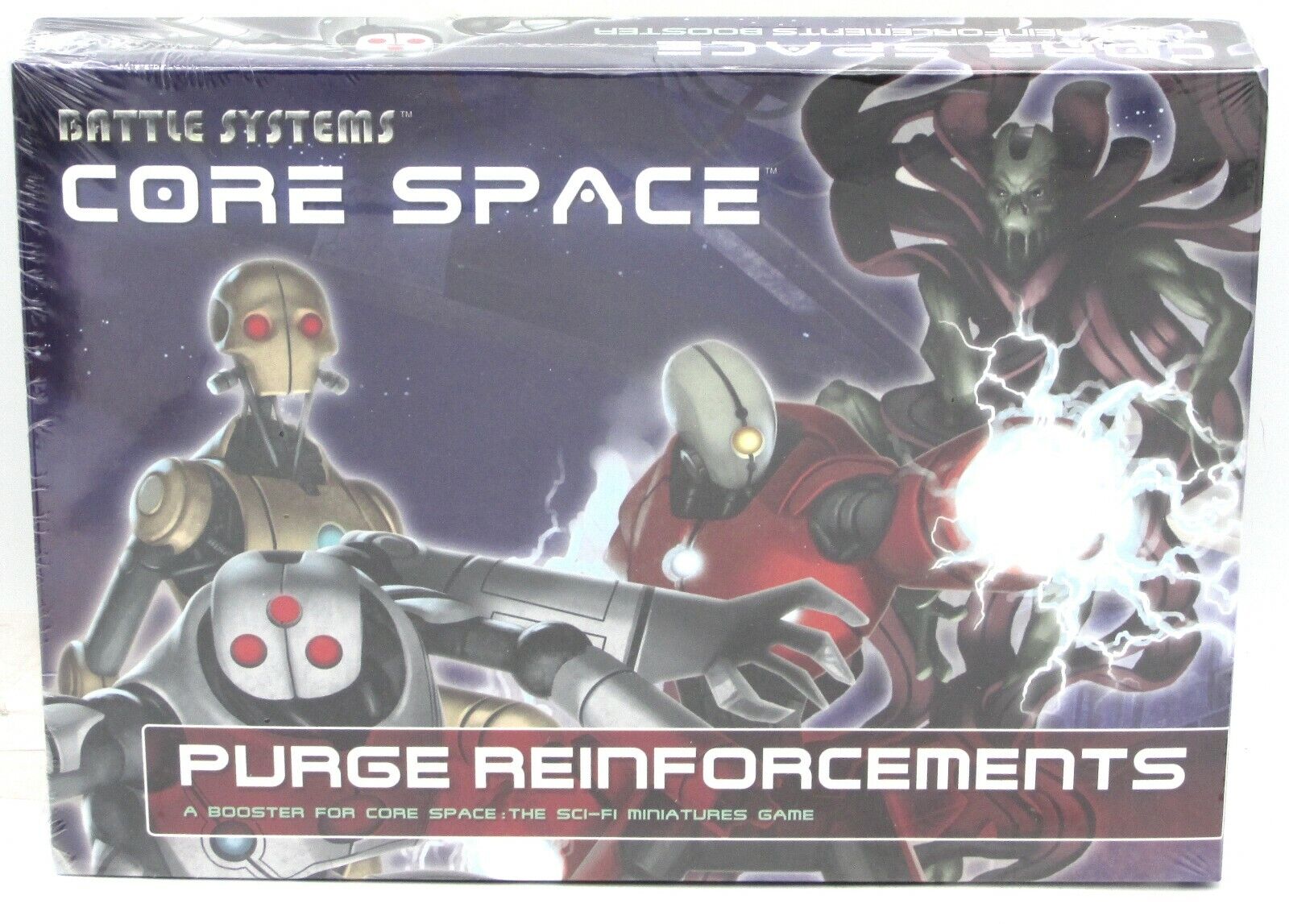The photograph captures a board game box at an angle, showcasing both the front and top sides. The rectangular box features striking artwork with various robots and aliens. On the top left, "Battle Systems" is written in silver text, with "Core Space" in white text below it. The central illustration displays four distinct creatures: a gold-colored robot with red eyes positioned at the top, a four-armed robot with three red eyes beneath it, a red-bodied robot with a gray head and a single yellow eye appearing to shoot a plasma ball to its right, and a green humanoid alien with black eyes and multiple scarves behind them. On the bottom of the box, within a maroon rectangle, "Purge Reinforcements" is prominently displayed in white font. The vivid depiction also includes spacecraft-like elements and what appears to be white lightning emanating from one of the robot's arms, enhancing the dynamic and futuristic theme.